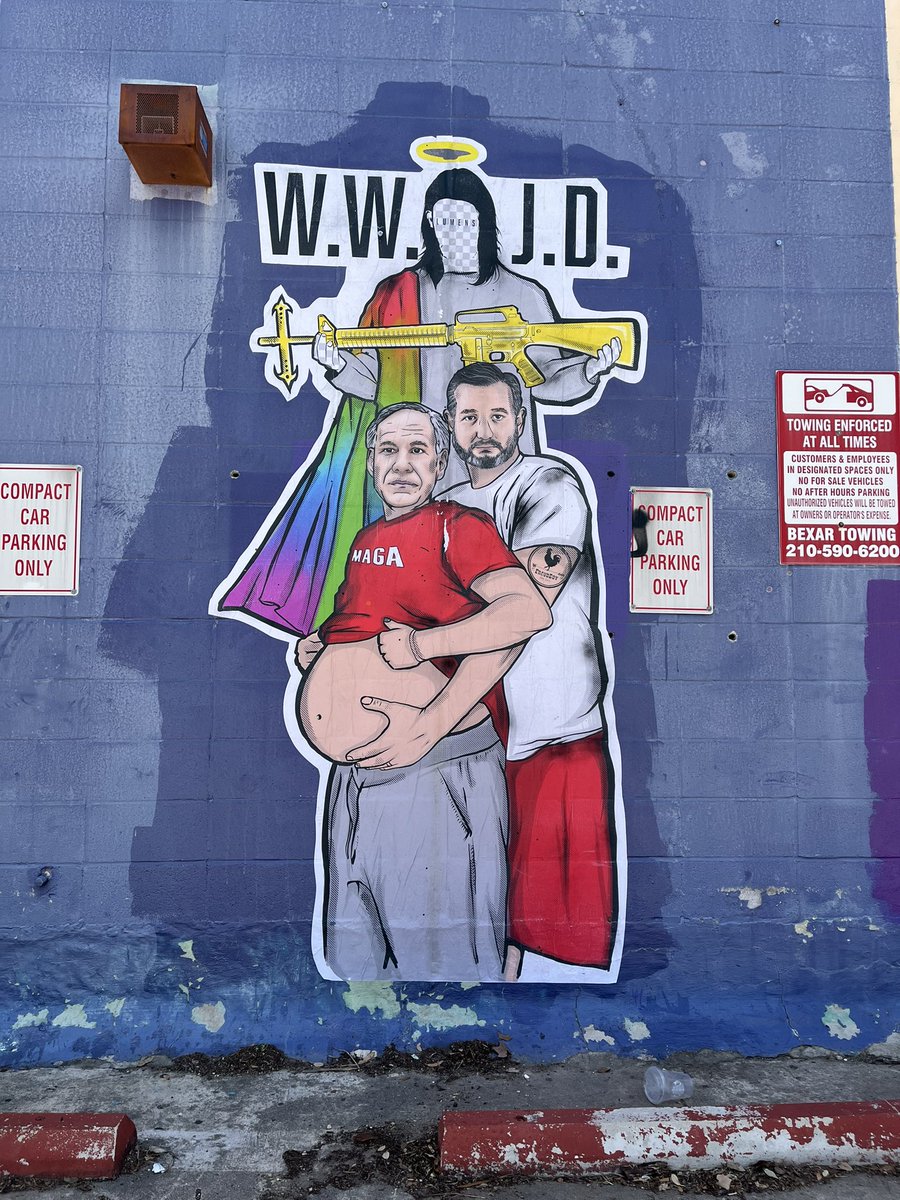The image depicts a striking mural painted on the side of a blue cinder block building, next to a parking lot. The mural features a larger-than-life figure resembling Jesus, adorned with a halo and a rainbow-colored shawl draped over his shoulder. He is holding a gun that has a cross at the end, and the letters "WWJD" are prominently displayed above him. The wall also has multiple signs, including two that state "Compact Car Parking Only" and another sign on the far right indicating "Towing Enforced at All Times."

In front of the mural stand two men in a pose reminiscent of traditional pregnancy photos. The man in the back, who is taller, has gray hair, a beard, and is wearing a white t-shirt with a rooster tattoo on his left arm and red basketball shorts. He is holding the round belly of the man in front, who is notably pregnant. This pregnant man, assumed to be a trans man, is older and is wearing a red shirt with the word "Mega" in white letters and light gray pants or shorts. The lower part of the mural is detailed with a red and white curb, accented by patches of moss and wear. The image captures a unique blend of contemporary social commentary and urban art.